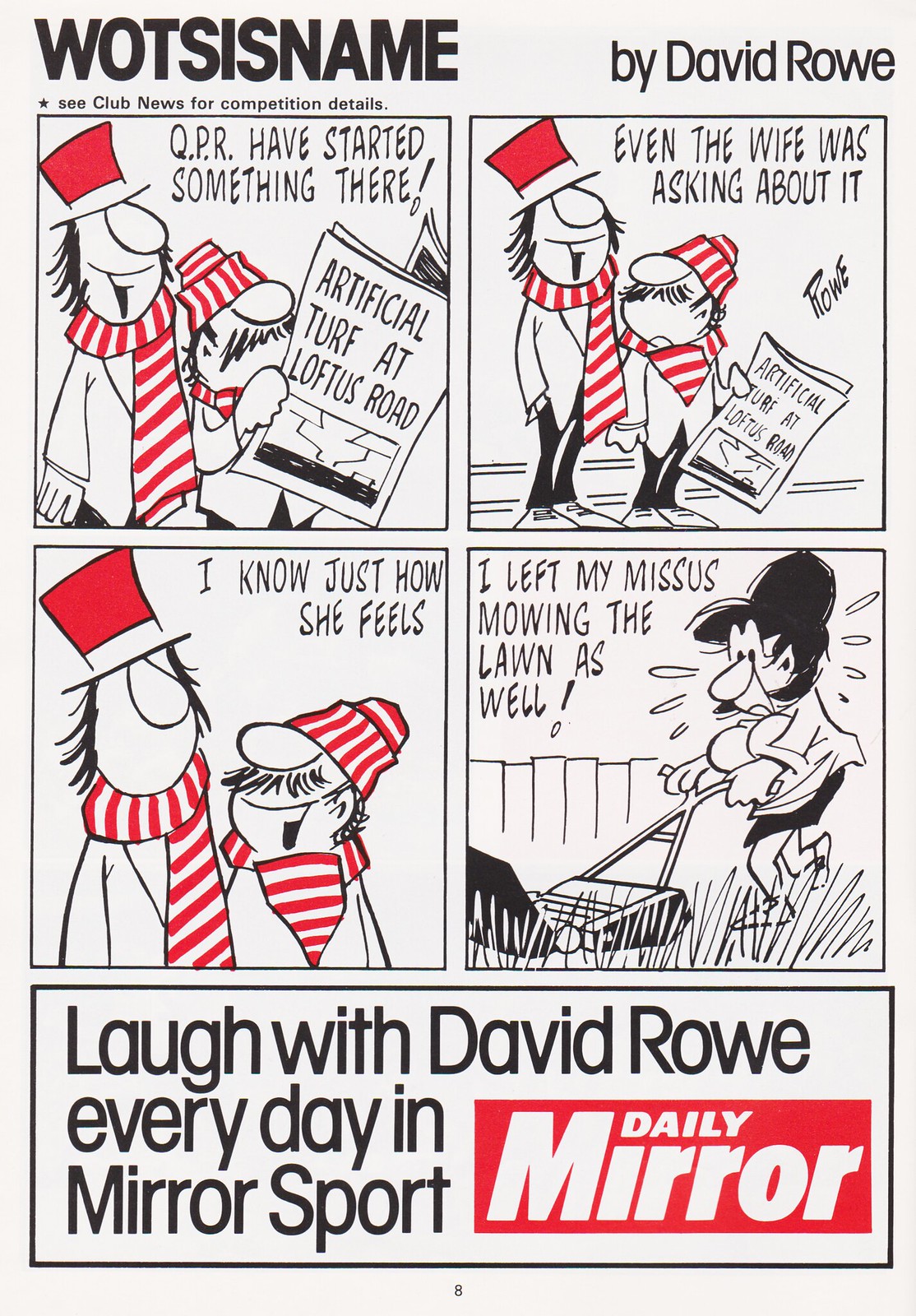The comic panel, "Wotsisname" by David Rowe, appears to be from a newspaper, specifically the Daily Mirror. It's a humorous four-panel black-and-white strip with red details. At the top, the title is prominently displayed in heavy black lettering with small print beneath it reading "Club news for competition details.” The comic depicts two caricatured men with large noses, wearing red and white-themed hats and scarves. In the first panel, one says, "QPR have started something there," referencing the headline "Artificial Turf at Loftus Road" on the newspaper they are reading. In the next panel, he continues, "Even the wife was asking about it." The third panel shows the second man replying, "I know just how she feels." Finally, in the fourth panel, he humorously adds, "I left my missus mowing the lawn as well," with an image of a happy woman mowing the lawn. Below the comic, there is an advertisement stating, "Laugh with David Rowe every day in Mirror Sport, Daily Mirror," accompanied by the red and white Daily Mirror logo.